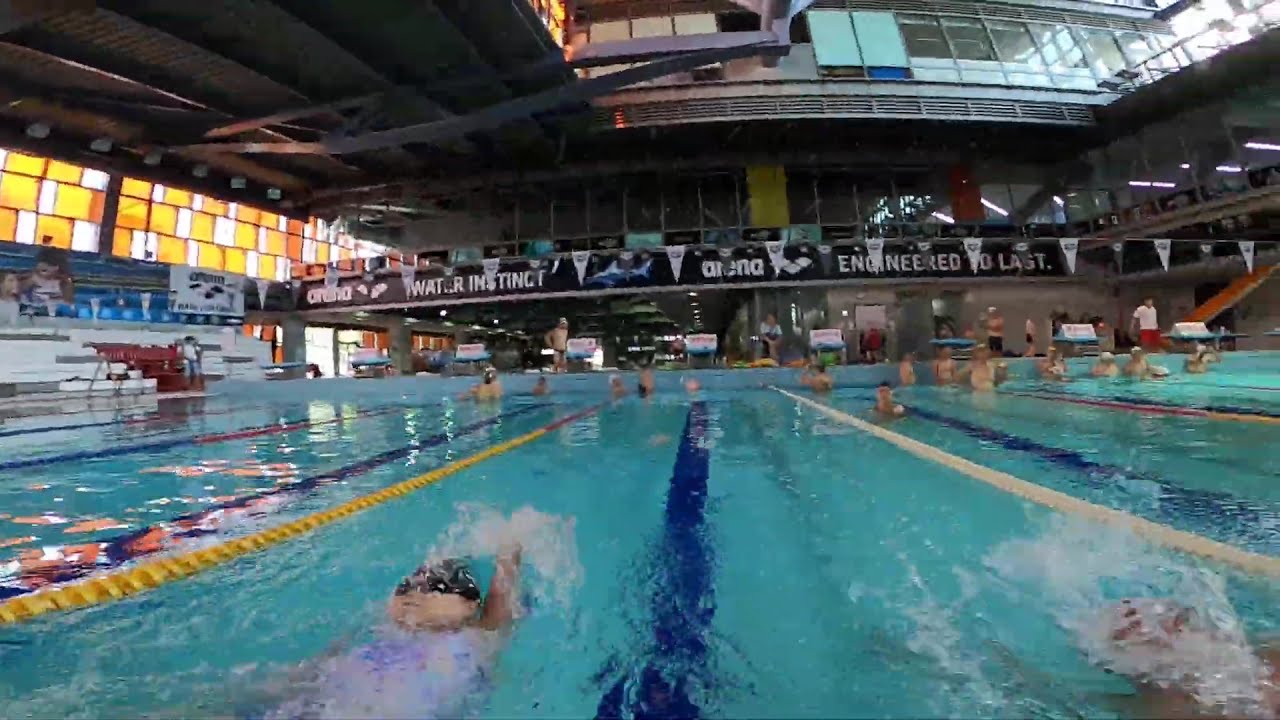This horizontally aligned rectangular image captures an indoor swimming meet, likely a relay competition, hosted in a multi-level building. The central feature is a pool with several lanes, demarcated by a yellow rope on the left and a white rope on the right. The pool stretches further across, though the image does cut off, subtly hinting at more lanes. In the pool, multiple swimmers, some appearing to perform backstrokes, are in action. 

At one end of the pool, several shirtless, somewhat blurred figures, who seem to be male, are gathered, perhaps waiting for their teammates to finish their leg of the relay. At the lower corners of the image, there are also swimmers who are likely participating in the ongoing relay. 

The backdrop reveals numerous windows on the upper level — some of them painted in stained glass hues of yellow, white, and orange, allowing light to filter through. Another striking feature is a banner stretched across the lanes in the center of the photo, adorned with small, upside-down triangular cutouts attached to a string. 

Above the pool, the banner reads "Engineered to Last," possibly an advertisement, adding an element of commercial presence within the venue. The color palette of the image consists of hues like light blue, dark blue, yellow, orange, red, black, white, and gray, accentuating the lively atmosphere. To the left, a few people occupy the stands, though they are sparse in number compared to the poolside activity. The overall ambiance suggests a vibrant indoor setting, brimming with competitive energy.